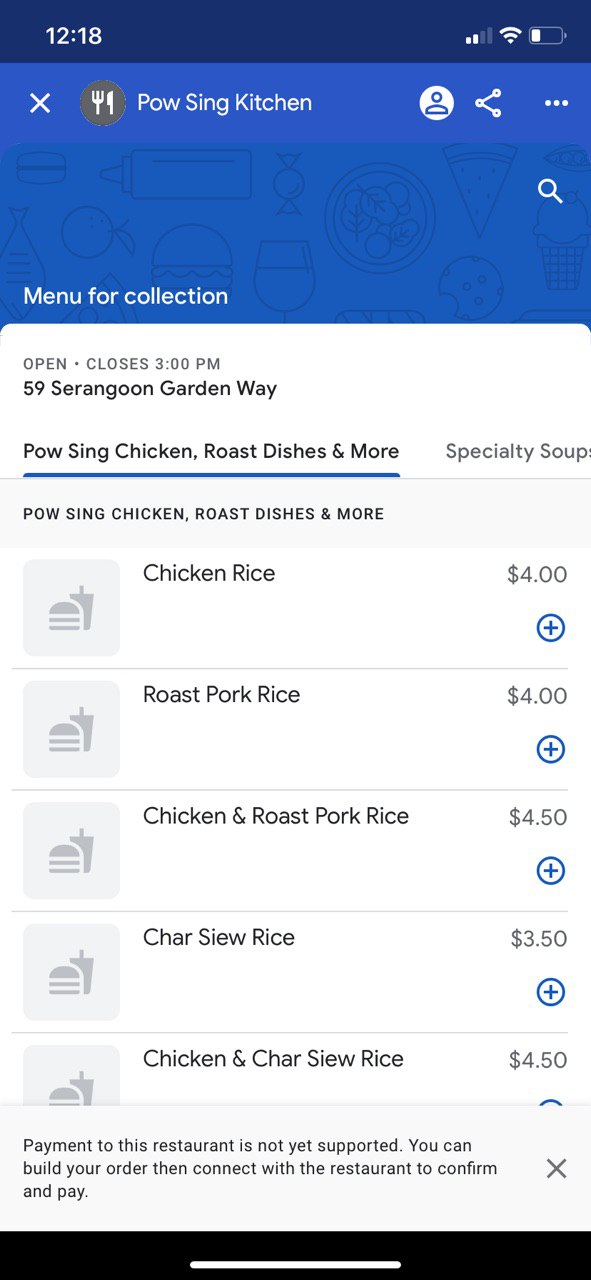This screenshot captures a detailed view of a mobile device, presumably an Apple iPhone, displaying an online menu for the restaurant Pow Sing Kitchen. The device's current time is 12:18 PM, with two bars of cellular service, full Wi-Fi connectivity, and a low battery. At the bottom of the screen, the familiar white line indicates the option to minimize the app, though it is unclear whether the app in question is Safari or a dedicated application.

In the upper section of the screen, a navigation bar includes an 'X' to exit the menu, along with icons for a profile, sharing options, additional settings, and a search magnifying glass. Central to the screen is the heading "Pow Sing Kitchen" accompanied by a gray circle with a white knife and fork icon. Below this header, the screen indicates that the restaurant is currently open, with hours listed until 3 PM, and provides the address: 59 Serangoon Garden Way.

The menu showcased is for both dine-in and take-out collection, with "Roast dishes and more" visibly selected from the categories. Another menu category, "Specialty soup," is present but currently grayed out, suggesting it is either unavailable or not selected. The items listed in the selected section include:

- Chicken Rice: $4 (with an add option via a plus sign).
- Roast Pork Rice: $4.
- Chicken and Roast Pork Rice: $4.50.
- Char Siu Rice: $3.50 (noted as S-I-E-W spelling).
- Chicken and Char Siu Rice: $4.50.

Each menu item has a designated spot for pictures, though no images are displayed at this time. It is also noted that direct payment through the menu interface is not supported; customers must build their order and then contact the restaurant to confirm and arrange payment.

In summary, this screenshot provides a clear and detailed look at Pow Sing Kitchen's menu via an iPhone, highlighting the operational status, various menu items with prices, and the current functionalities and limitations of the ordering system.